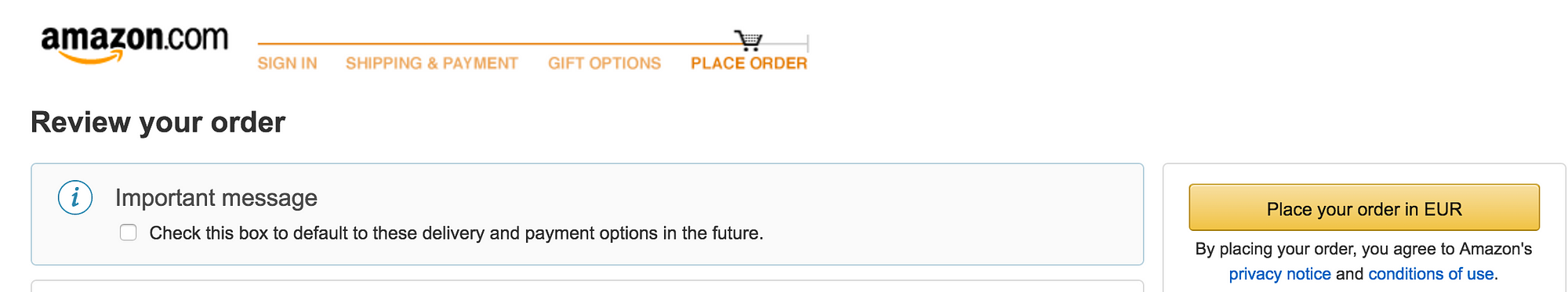This is a cropped, rectangular, and very thin screenshot of the Amazon.com "Place Order" page. The top left corner prominently displays the Amazon.com logo. To the right of the logo is an orange navigation bar, which includes a shopping cart icon towards its right end, situated just above the "Place Order" button.

Under the orange navigation bar, there are four progress points indicating the steps of the checkout process. The first point on the far left reads "Sign In," followed by "Shipping and Payment," then "Gift Options," and finally, "Place Order" in bold orange letters, signifying the current step.

Beneath these progress points, on the left side, the text "Review your order" appears in bold black font. Directly below, a large gray rectangle encapsulates an alert message. This message features an eye icon in the top left corner, next to the text "Important Message." Below this, the alert instructs users to "Check this box to default to these delivery and payment options in the future," with a small checkbox provided to the left.

On the right side of the gray rectangle, there is a small box section which includes a large yellow bar. Inside the yellow bar, it prompts users to "Place your order in Euros." Underneath this bar, there is additional text: "By placing your order, you agree to Amazon's privacy notice and conditions of use." The terms "privacy notice" and "conditions of use" appear in bold, small blue print for emphasis.